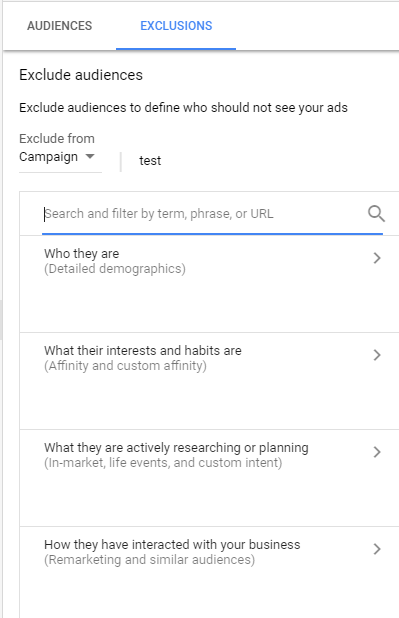A screenshot of an advertising platform’s settings page, specifically showcasing the "Audiences and Exclusions" section. At the top of the page, the tab "Exclusions" is highlighted, indicating that the user is currently setting up exclusions for their ad campaign. The description at the top of this section reads, "Exclude audiences to define who should not see your ads," guiding the user on the purpose of the exclusions.

Underneath, there is an option labeled "Exclude From," accompanied by a drop-down menu from which "Campaign" is currently selected. Adjacent to this is another field labeled "Test," though its exact function is unclear. Below these fields, there is a search box with a placeholder text that says "Search and filter by term, phrase, or URL," where users can input specific criteria for exclusion.

Further down, the page is divided into detailed categories for audience exclusion. These categories include:

1. **Who they are**: This section entails "Detailed Demographics," with an arrow indicating more options for selection.
2. **What their interests and habits are**: Contains "Affinity and Custom Affinity" audiences, again with an arrow for further details.
3. **What they are actively researching or planning**: Includes options like "In-Market," "Life Events," and "Custom Intent."
4. **How they have interacted with your business**: Pertains to "Remarketing and Similar Audiences."

An example scenario elaborates that if a user wishes to exclude pregnant individuals from their campaign, they would specify "pregnant" under detailed demographics, and include interests like "baby items" or "having a baby" under the relevant sections. Additionally, they may exclude users who have previously searched for or interacted with "baby items" on their website.

This comprehensive control allows advertisers to precisely tailor their target audience by excluding specific groups, ensuring the ads reach the most relevant viewers.